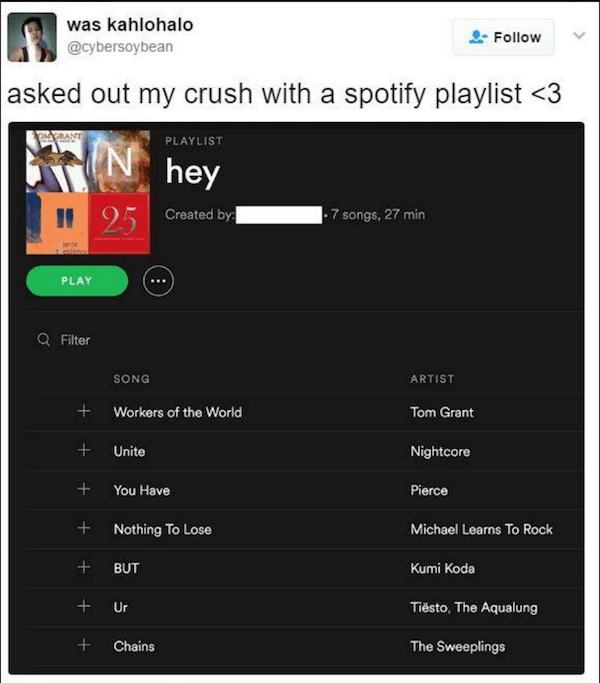This image depicts a section of a social media profile. In the top left corner, there is a profile picture of a white female with a short black haircut, wearing a black strap-top. The light highlights the right side of her face and her shoulders are exposed. Next to the profile picture, the username "K-A-H-L-O-H-A-L-O" is displayed, followed by the handle "@CyberSoybean."

On the right side of this section, there is a blue "Follow" button with a person icon and a drop-down arrow next to it. Below this is a heading that reads "Asked out my crush" accompanied by a Spotify playlist icon and an arrow pointing to the left with the number "3."

Central to the image is a large black box showcasing an album cover. To the right of this cover, the heading "Playlist" is displayed. Underneath, bolded in white text, is the title "hey" in lowercase, followed by the note "created by" (which is whited out). It indicates the playlist contains "7 songs, 27 minutes."

Below the album cover, there is a "Play" button, beneath which is an option to filter songs. Each song title is listed along with the corresponding artist on the right-hand side.